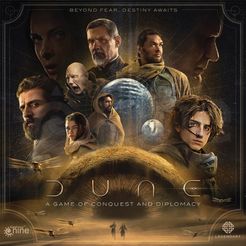This is a detailed description of a promotional poster for the tabletop game "Dune: A Game of Conquest and Diplomacy," which features imagery from the movie "Dune." The poster is square-shaped and prominently showcases various elements associated with the cinematic adaptation.

At the top of the poster, the text reads, "Beyond Fear, Destiny Awaits," setting a tone of epic adventure. Below this text are images of several characters from the film, including Timothee Chalamet, Oscar Isaac, and Josh Brolin, among others. These characters are somewhat dark and shadowed, and their faces are arranged in a way similar to traditional movie posters.

In the center of the poster, two planets are depicted, with one larger and one smaller, symbolizing the interplanetary setting of the "Dune" universe. Beneath these planets, the word "DUNE" is prominently displayed in large letters, and directly underneath it, in smaller font, is the subtitle "A Game of Conquest and Diplomacy."

At the bottom of the poster, two small, somewhat blurry human figures are seen running away from a massive sandworm, a central element of the "Dune" mythology. The sandworm's mouth, resembling a pupil, adds a menacing and dramatic flair to the scene. The imagery effectively combines elements of the film with the board game, creating a visually compelling advertisement.